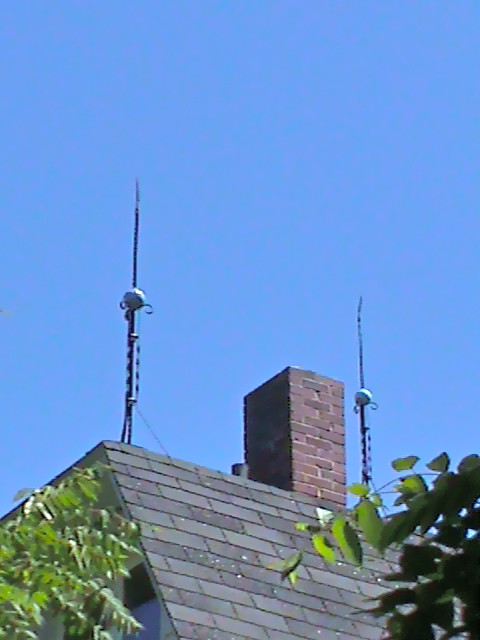This image captures a bright, clear day with a crystal blue sky devoid of clouds. At the center of the scene is a slanted rooftop composed of dark and light gray rectangular shingles. Crowning the roof at its peak is an old, reddish-brown brick chimney. Flanking the chimney are two black poles, likely antennas or lightning rods, each featuring a round white disc at the top. To the left of the rooftop, a lush green tree is visible just below the roofline, while on the right, green branches with leaves extend and frame the scene against the sky. The overall composition creates a serene and picturesque outdoor setting, with the vivid colors of the sky and greenery contrasting against the earthy tones of the roof and chimney.